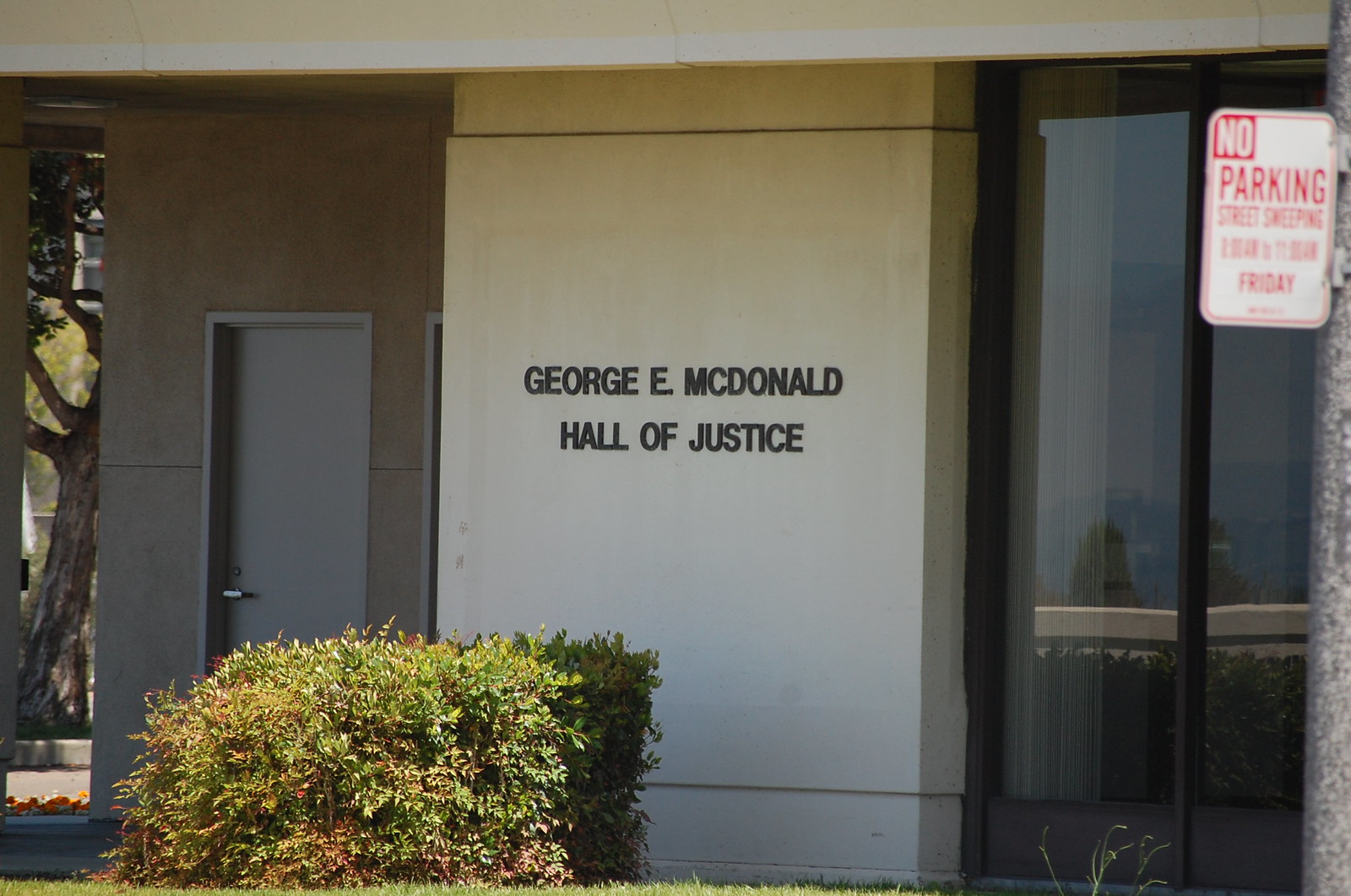This photo captures the front facade of a building, prominently featuring the name "George E. McDonald" and "Hall of Justice" in black letters centered on a smooth, light beige wall. Below the sign, there's a well-maintained, square-shaped bush basking in the sunlight, which illuminates the green grass in front. To the left, the wall recedes slightly, revealing a couple of subtle, dark-colored beige doorways and a nearby tree. On the right side, there are floor-to-ceiling glass panes with dark brown trim, reflecting the sunlight. At the very edge of the photo, a pole displays a red and white no parking sign, adding to the everyday scene of this seemingly courthouse-adjacent exterior.